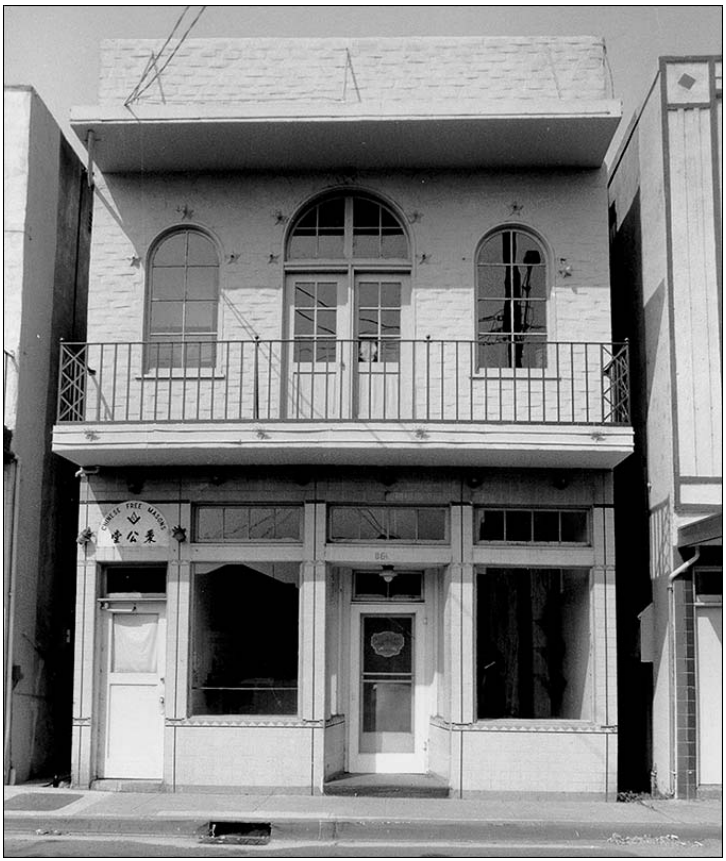This black-and-white photograph depicts the exterior of an older, two-story building, likely from the mid-20th century and situated on a densely populated city street, possibly reminiscent of New Orleans. The building, which appears to house two separate businesses, spans the entire frame of the image and features minimal space between adjacent buildings, barely wide enough for a person to pass through.

The ground floor serves as a storefront, characterized by two large plate glass windows flanking two primary entry doors. The door on the left has a semi-circle sign above it, partially legible with English and Chinese characters indicating "Chinese Freemasons." However, some parts of this sign are unclear. The door on the left also has a curtain covering its glass panel. The shopfront windows are bare, hinting that the businesses might be vacant.

The upper floor features a metal-balustraded balcony spanning the width of the building, accessed by double French doors with a semi-circular transom window above them. On either side of these doors are two arched windows with clear-story design. The roof, visible in the photograph, is made of brick and includes an additional awning extending from it.

Overall, the architecture and details such as the iron railings, arched windows, and French doors, encapsulate an aged elegance, drawing a picture of historical significance in a bustling urban environment.